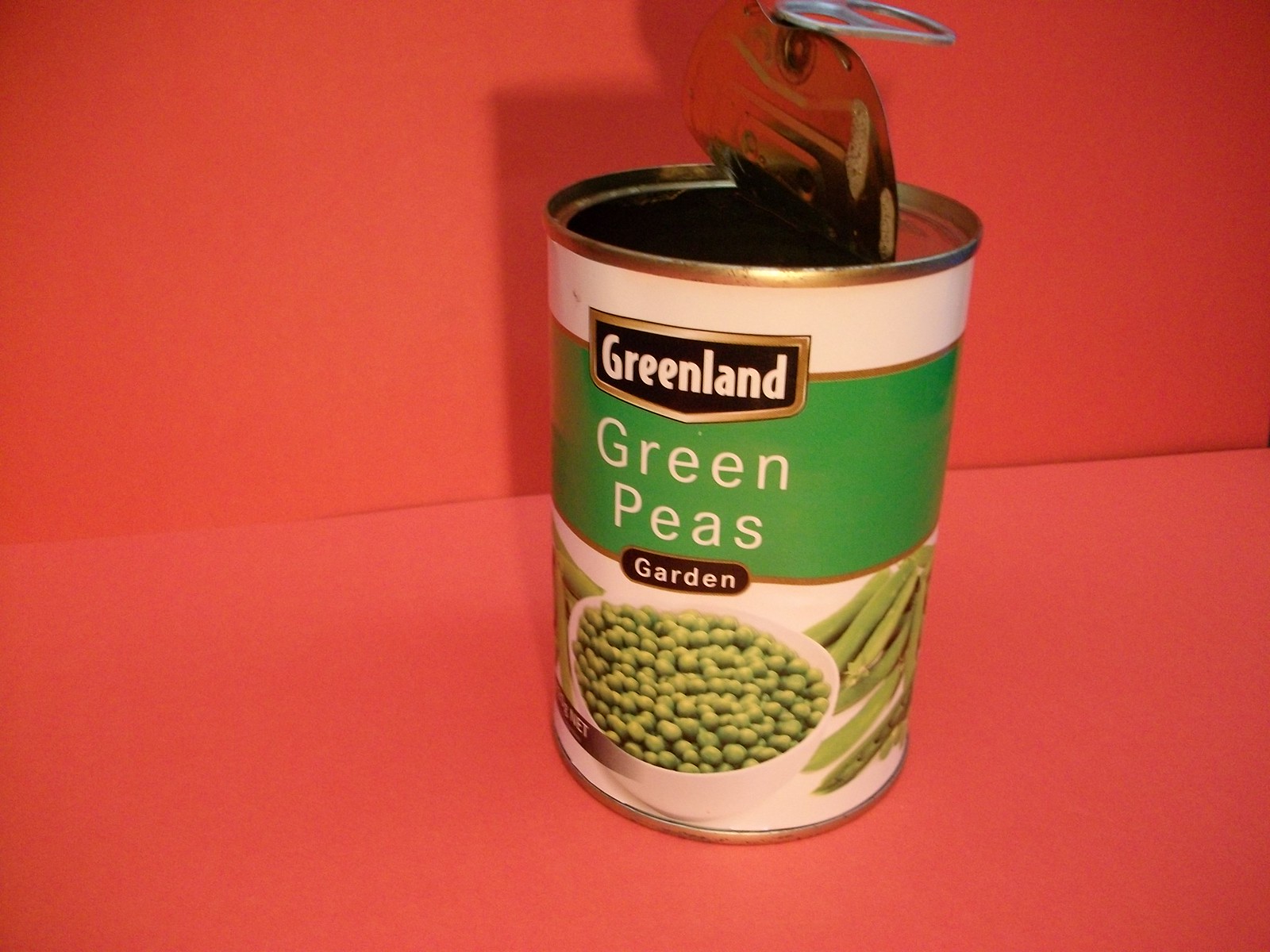This photograph showcases a tin can of peas set against a vibrant red background, resting on a matching red surface. The can features a convenient pull-tab pop-top, which has been partially opened, revealing its contents. The can is adorned with a white paper label, highlighted by a green stripe encircling it. Prominently displayed on the label are the words "Greenland Green Peas Garden," along with a vivid photograph of a bowl filled with green peas, accompanied by scattered pea pods, emphasizing the freshness and quality of the product.